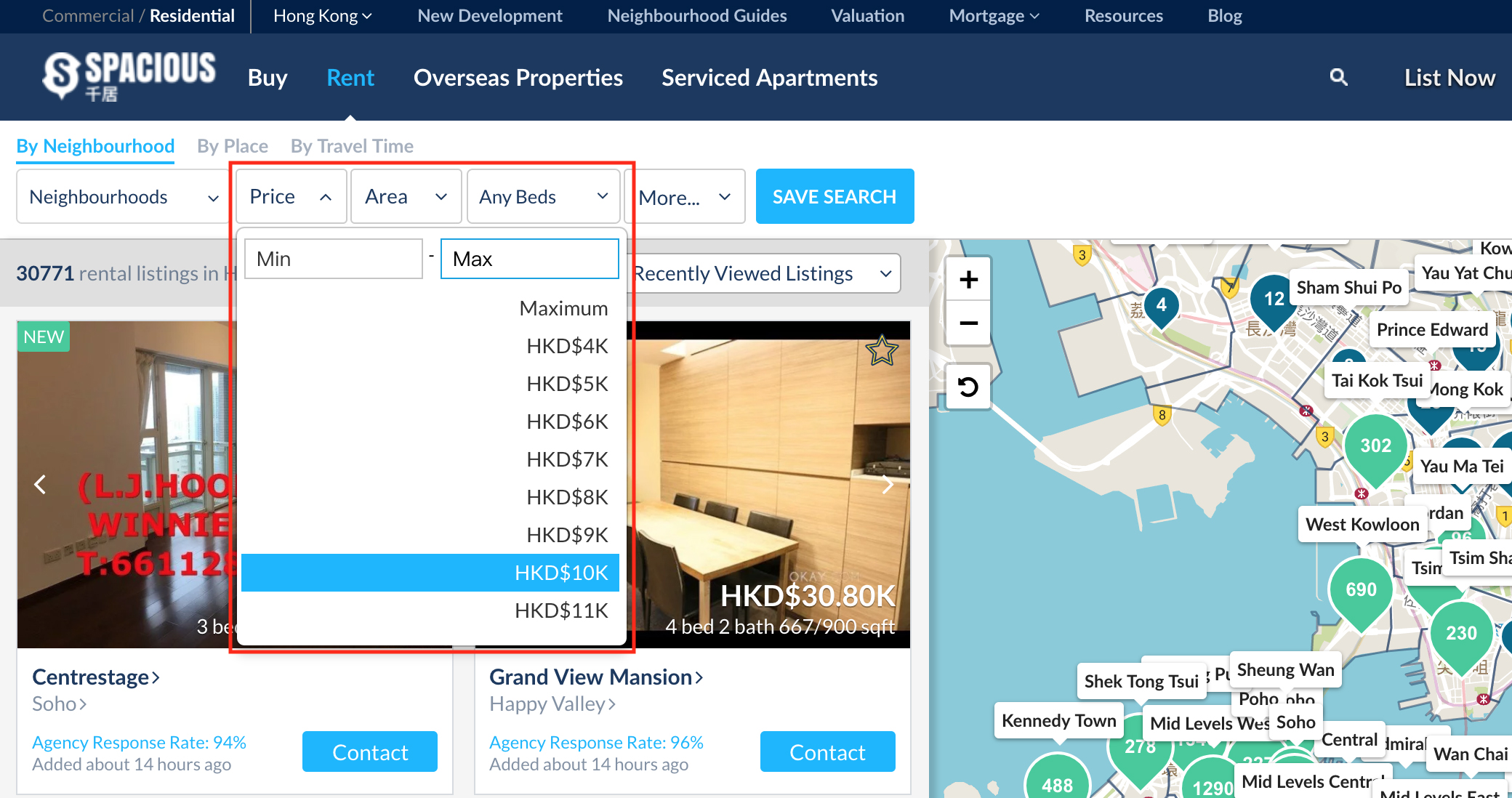The image features a visually structured layout with distinct sections primarily utilizing varying shades of blue and white. 

At the top, there is a dark blue banner containing text that is too small to be legible. Directly below, a slightly lighter blue rectangle features a prominent "S" outlined in white, followed by the word "spacious" also in white. Adjacent to the word "spacious," phrases such as "buy in," "overseas properties," and "service departments" are displayed, each alternated in white and blue text. 

On the right side of this section, a magnifying glass icon accompanies the words "list now." Underneath this area, there is another white background section prominently displaying the phrase "buy neighborhood" in blue text, which is underlined. Next to it are options labeled "buy place" and "buy travel time."

Further below, the phrase "neighborhood" appears in black font under the "buy neighborhood" line. This is followed by a red-outlined rectangle containing a white rectangle within it, showing fields labeled "price," "area," "any beds," "min," and "max."

Beneath these fields, additional text is presented along with images partially obscured by the white rectangle. These images appear to depict various apartments, with what seems to be the names of the apartments below them. 

Each image is coupled with a blue rectangle labeled "contact," and towards the right-hand side, a map is displayed.